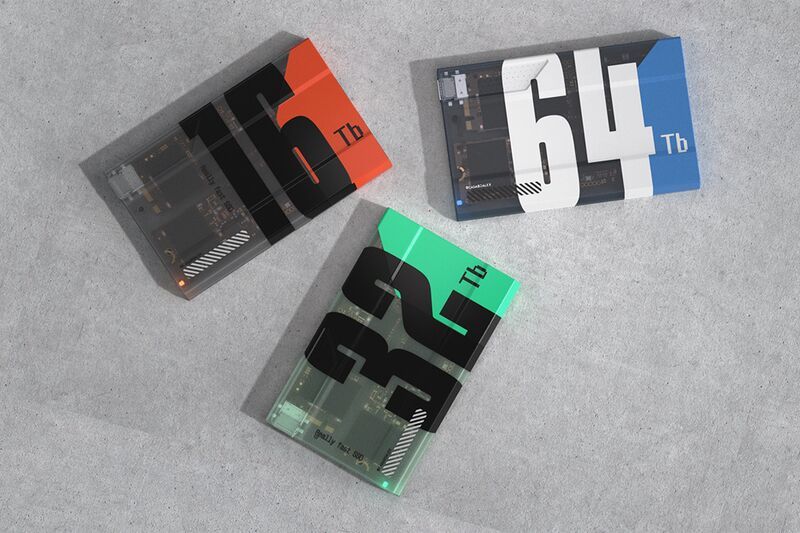The photograph features three rectangular SSD-style hard drives resting on a light gray surface, each casting a shadow. The drives are housed in translucent plastic casings that reveal the intricate circuitry inside. The top left drive is marked "16TB" in bold black lettering and is accentuated by a red border on its right side. Below it, the drive showcases a "32TB" capacity in bold print on a translucent green case, highlighted by a bright green border. Finally, the top right drive displays "64TB" in bright white bold font, enclosed in a translucent blue case with a striking blue border.